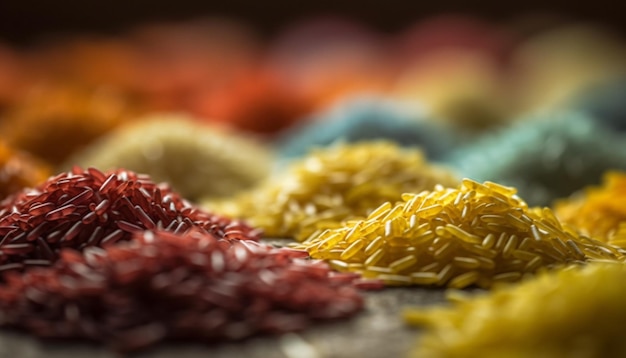The photograph showcases an arrangement of small piles of differently colored rice, set against a black surface. In the foreground, the sharp focus highlights a central pile of yellow or golden rice with glossy kernels, suggesting they might be plastic or artificially colored. To the left of this pile is a cluster of red rice, equally detailed. The image further extends into a blurred background, displaying additional piles in various colors, such as light blue, orange, green, and even pink. The out-of-focus background makes it difficult to discern individual grains in those distant piles. The overall impression is of vividly colored grains, possibly dyed rice, arranged in small, distinct heaps, with the foreground emphasizing the yellow and red varieties.